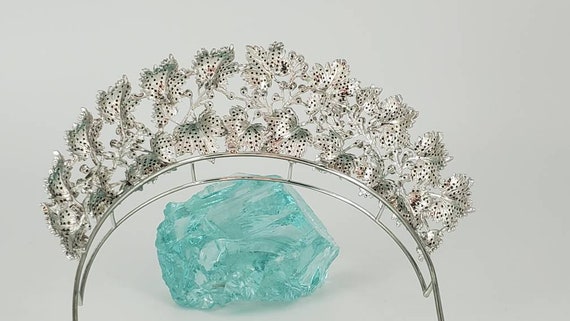The photograph depicts a striking arrangement set against a plain light gray background. At the forefront is a large, uncut crystal rock formation, transparent and pale aqua blue, reminiscent of the ocean's hue. The crystal, irregular in its natural shape, is approximately the size of a hand. Gracefully arching over and partially resting on the crystal is an ornate silver tiara with a thin, stainless steel-like frame designed to resemble a crown. This elegant tiara is adorned with intricate metal flowers and leaves, each embellished with small black dots that line their petals and leaves. The composition highlights the delicate interplay between the crystalline structure and the refined metallic embellishments of the tiara, creating a captivating and harmonious visual.